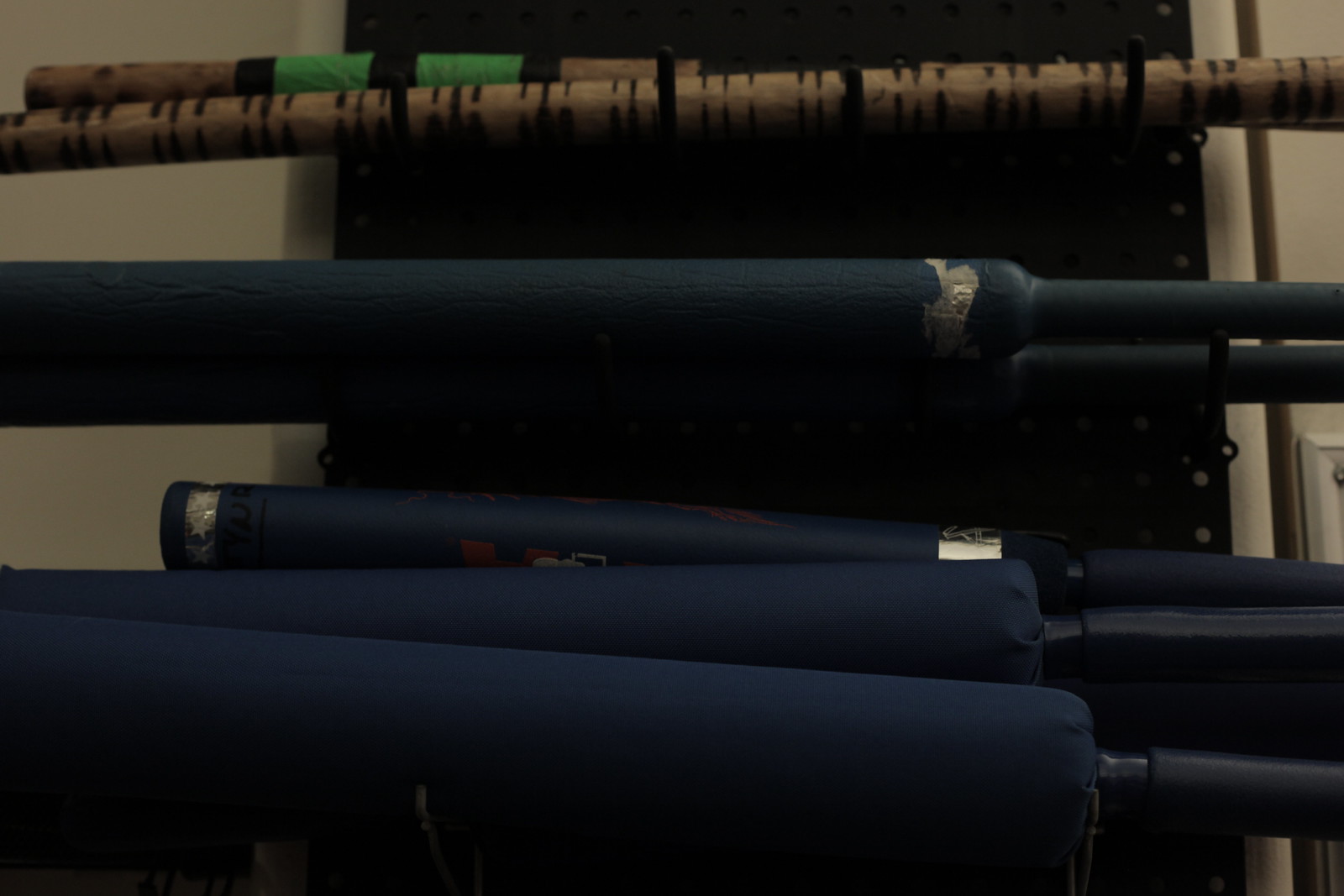This image features several elongated objects resembling umbrellas or rolled-up fabrics. Arrayed vertically, these items come in various colors and designs, including navy blue and beige with blue stripes. They are reminiscent of outdoor furniture umbrellas that can be unwrapped to provide shade. The objects appear cushioned, with some displaying black line designs that run up and down their lengths, similar to decorative or functional rods. Positioned against a grate-like black metal backdrop, they create a striking visual against an off-white plaster wall. These objects also feature handle-like elements, further suggesting a utilitarian design, possibly related to handheld or collapsible devices.